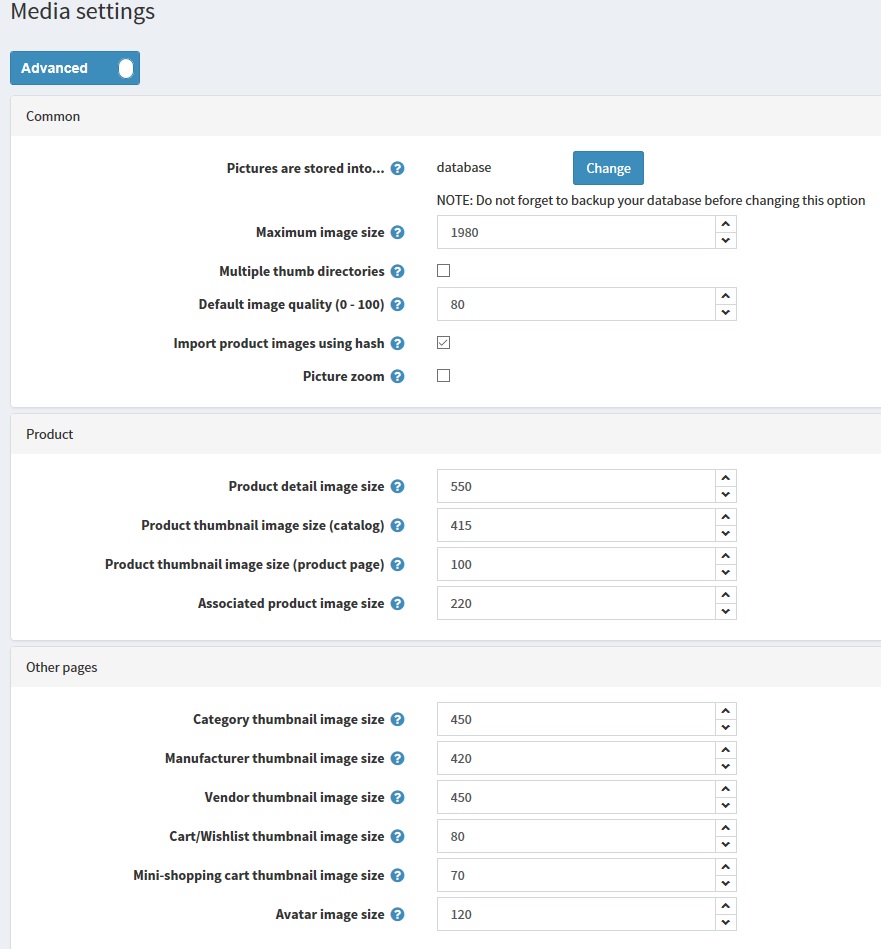**Detailed Caption:**

The image depicts a detailed settings page from a website, viewed on a laptop screen. The top part of the image features a very faint pale blue bar stretching across the width. In the upper left corner, black text reads "Media Settings." Directly below, there's a long blue clickable bar labeled "Advanced," featuring a white up-and-down oval icon on its far right.

Below this, a long gray bar appears with the black text "Common" on the left side. The central section of the page includes various adjustable settings, displayed as a large rectangular white area with numerous clickable options. Midway through, there's a black text label "Pictures are stored into," accompanied by a blue circle with a white question mark inside, followed by more black text "Database." To the right, there's a blue box labeled "Change" in white letters. 

Below the storage section, a series of options follows, each accompanied by blue circles with white question marks to their right. These options include:
1. Maximum Image Size
2. Multiple Thumb Directories (with a checkbox next to it, currently unchecked)
3. Default Image Quality (0 to 100)
4. Import Product Images Using Hash
5. Picture Zoom

To the right of these settings, a black text note reminds users: "Note: Do not forget to back up your database before changing this option." Below this note, there's a white box set to "1980" with up and down arrows for adjustment. 

Adjacent to the "Multiple Thumb Directories" setting is another white box marked "80" with similar adjustment arrows. A gray checkbox with a checkmark and an unchecked square box follow below. 

Further down, another gray bar labeled "Products" in the upper left corner introduces a new section. Again, the blue circle with a white question mark is present, along with four settings:
1. Product Detail Image Size
2. Product Thumbnail Image Size (Catalog)
3. Product Thumbnail Image Size (Product Page)
4. Associated Product Image Size

Each setting has a corresponding adjustable white box on the right. The top box is set to "550," followed by "415," "100," and "220" respectively.

Another faint gray separator introduces the "Other Pages" section. In the upper left, black text reads "Other Pages," followed by six rows of settings, each with the standard blue circle and white question mark:
1. Category Thumbnail Image Size
2. Manufacturer Thumbnail Image Size
3. Vendor Thumbnail Image Size
4. Cart/Waitlist Thumbnail Image Size
5. Mini Shopping Cart Thumbnail Image Size
6. Avatar Image Size

Accompanying these settings, on the right, there are adjustable white boxes with the following numbers:
1. 450
2. 420
3. 450
4. 80
5. 70
6. 120

Each adjustable box features up and down arrows to modify the values as needed.